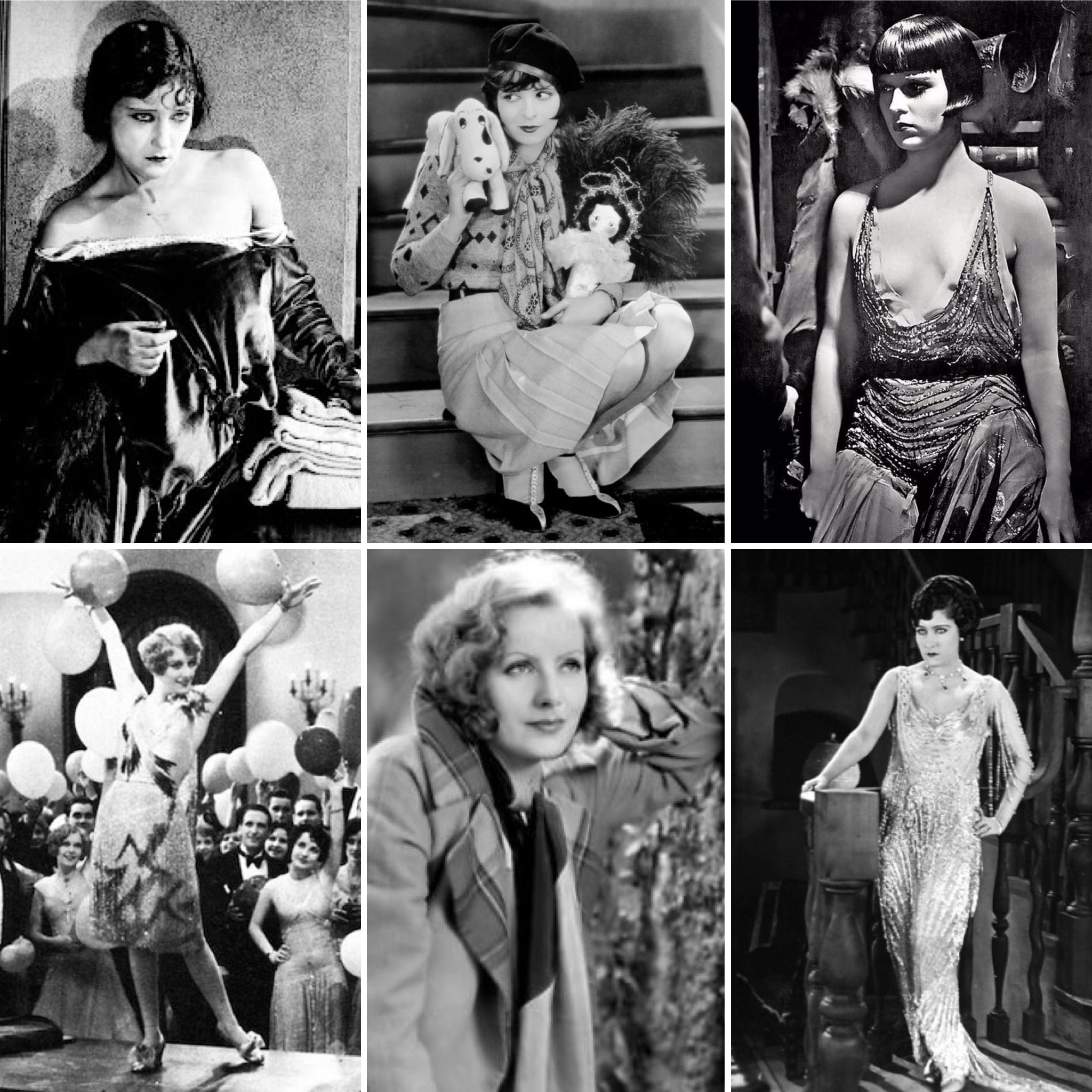This is a detailed collage of six photographs, arranged in a three-by-two grid, all showcasing what appears to be the same actress in various outfits and settings. In the top left image, she sports a pixie cut with greasy-looking black hair, adorned in an off-the-shoulder black dress, exuding a serious and sultry demeanor. The middle image in the top row features her with a lighter hair color, wearing a knee-length skirt, patterned shirt, and a cap, while holding stuffed animals. Completing the top row, she dazzles in a shimmery, low-cut, Gatsby-esque dress, her short bob haircut complementing the glitzy appearance.

On the bottom left, she appears exuberant, waving her arms in the air amidst a festive atmosphere, possibly a birthday party, with balloons in the backdrop. Next, in the middle image of the bottom row, she dons a stylish coat with a scarf, notably highlighted with a Burberry-like logo, casting a distant, contemplative gaze. The collage concludes with the bottom right image, where she is elegantly clothed in a floor-length, silver sequin gown, showcasing intricate beaded pleats on the shoulders, and once again, emanating a sexy allure. The collective imagery succinctly captures her versatility and dynamic presence.